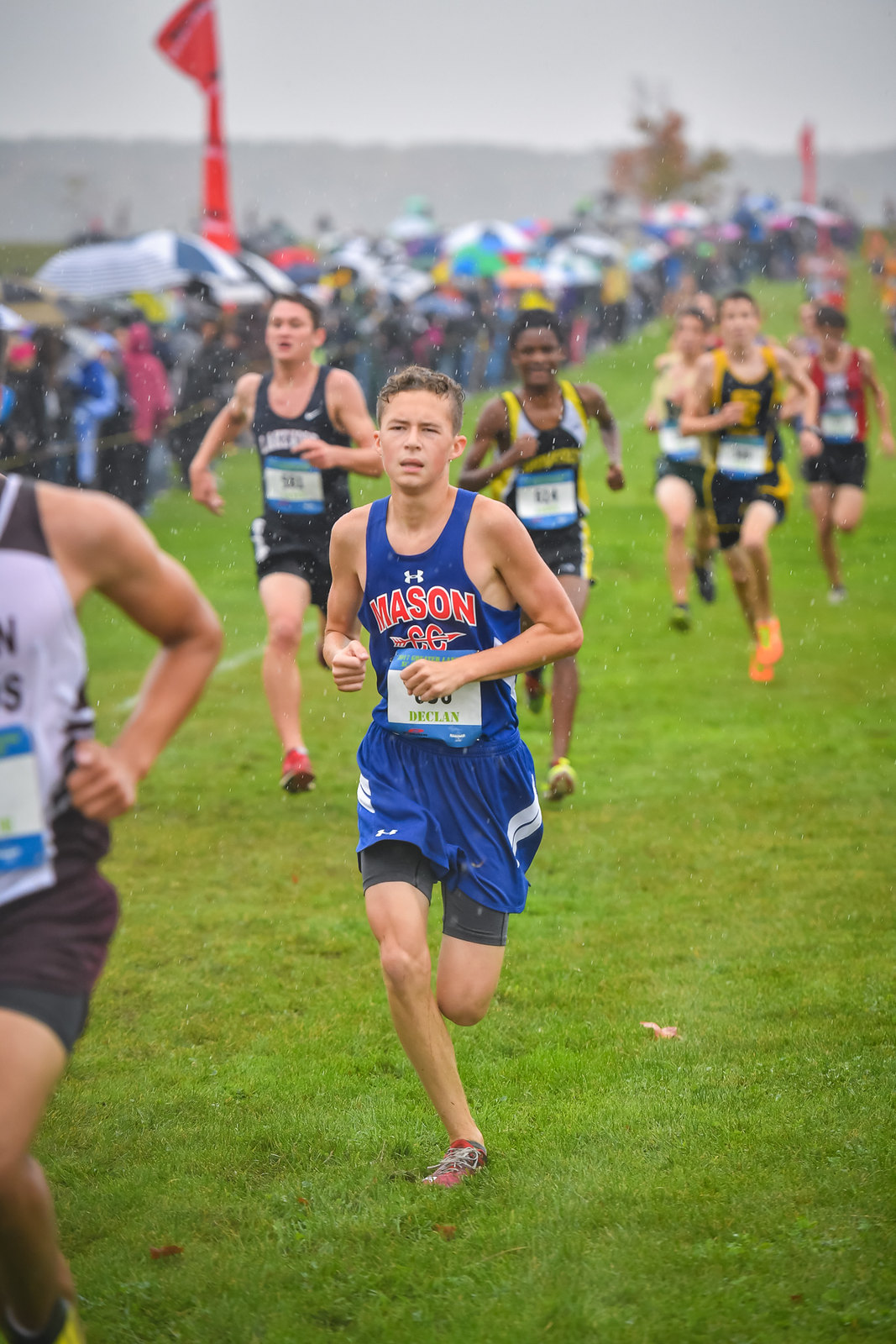This photograph captures the intensity and atmosphere of a high school cross-country race taking place on a rainy day. At the forefront, a determined male runner, clad in a blue Under Armour tank top and matching blue shorts with white stripes, stands out. His tank top bears the red lettering of “Mason,” indicating the school he represents. He pushes forward on the grassy terrain, visible raindrops adding to the blurred urgency of the scene. His race bib, partially obscured by his hand, hints at the competitive nature of the event.

Surrounding him, seen in various stages of exertion, are 8-9 fellow competitors, some in red, yellow, and orange shoes, each with their own race numbers pinned to their shirts. The vivid colors of their footwear punctuate the otherwise gray and gloomy atmosphere, with a sky pregnant with rain clouds adding a dramatic backdrop to the race.

Spectators line the side of the racecourse, their faces partially hidden under the umbrellas and makeshift covers they hold to shield from the rain, fervently cheering on the runners. The scene stretches back to reveal a crowd of at least 15-20 people, all blurred into the wet and overcast ambiance of the day. White marker flags guide the runners as they navigate the course, emphasizing the organized, yet grueling nature of the race held under the relentless drizzle.